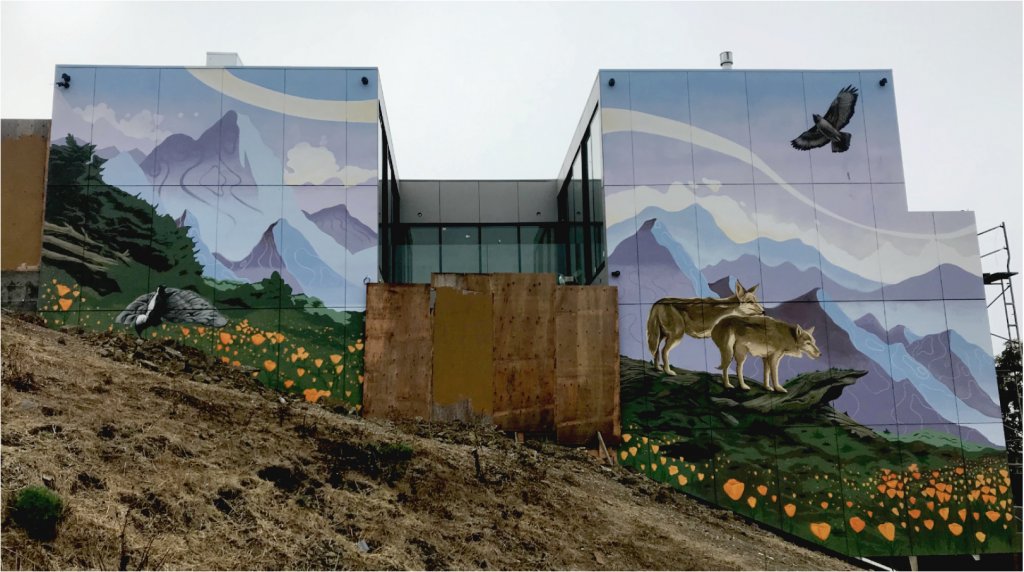The image depicts a modern cubic-shaped building situated on a brown or tan hillside, with patches of green grass and yellow flowers scattered around. The building features three main compartments: two sides facing the viewer and a recessed central section with large glass windows, partially covered with wooden or metallic boards. Both visible side walls of the building are adorned with detailed murals. On the left wall, a mural showcases a lush green landscape with vibrant yellow flowers, blending seamlessly into the real greenery surrounding the structure. The right wall displays a detailed scene of gray and tan wolves standing on a rock-strewn hillside, with a black bird soaring through the sky above. In the middle section, windows allow a glimpse inside, and silver stands with black platforms suggest ongoing artistic work. The background features a range of purple and gray-blue mountains under a whitish-gray sky punctuated by white clouds. The overall ambiance is serene, capturing the harmony between the building and its natural and painted surroundings.